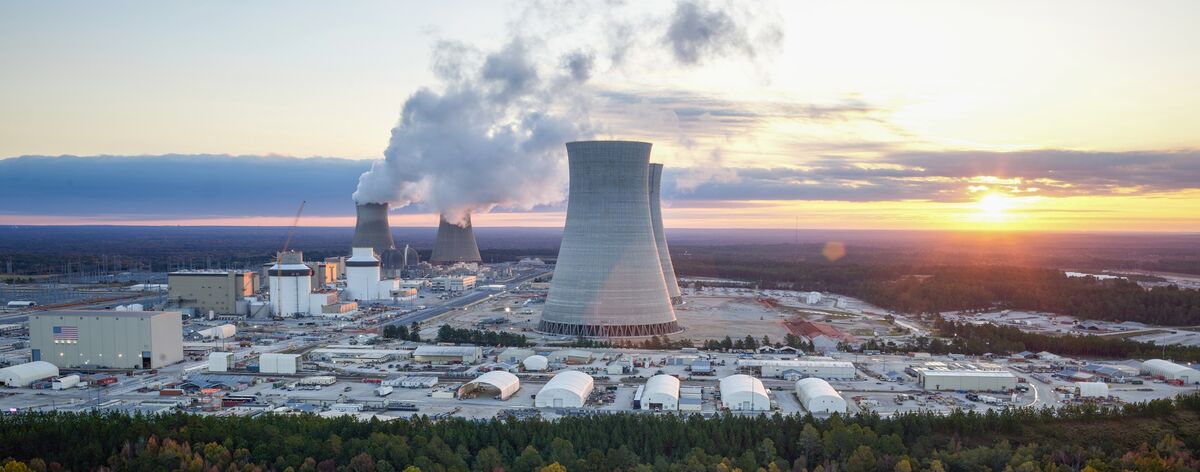The image depicts an expansive manufacturing site captured from an aerial perspective, featuring four prominent white power plant towers with rounded, tapering tops. Two of these towers are billowing thick clouds of smoke into the sky. Encompassing the area are numerous smaller structures, predominantly white with some beige, scattered across the site. On the left side, a notable warehouse with a United States flag is visible, accompanied by four light bulbs positioned below it. In the foreground, rows of green trees form a lush boundary, while in the distance, a setting sun casts an orange tint over the horizon. Additionally, a body of water and scattered clouds add to the landscape’s depth, creating a vivid and detailed portrayal of this large industrial facility.